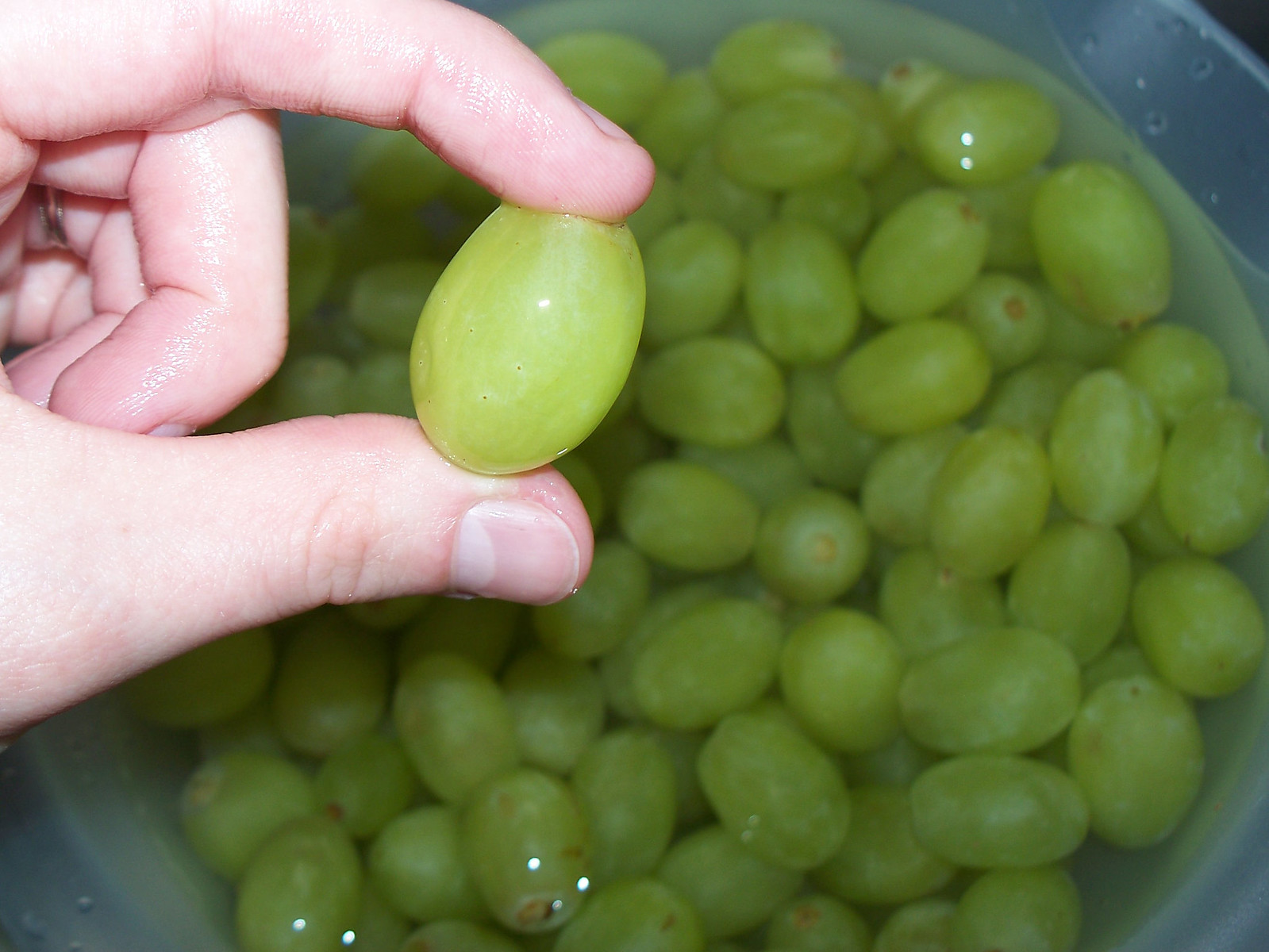In this close-up photograph, a person's hand with a light complexion and a ring on one finger is holding a large green seedless grape between their thumb and forefinger, presenting it up to the camera. Just below the hand, there is a white bowl with a blue rim, filled with hundreds of green grapes immersed in water for rinsing. The grapes are densely clustered together and some of them show small white dots, possibly due to issues with the film or flash. The bowl is filled up to the brim, and the scene focuses on the preparation process of cleaning the grapes, readying them for consumption.